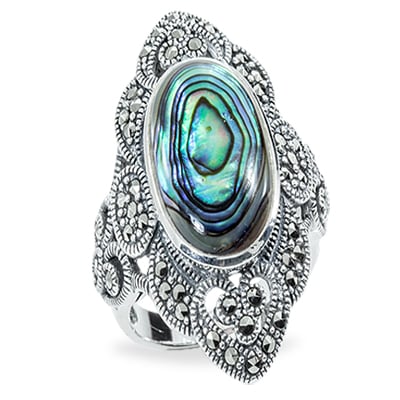The image features a single, silver-colored ring set against a completely white, unadorned background. The ring is highly artistic and antique-looking, with intricate carvings and ornate designs encompassing its band. Embedded within the band are tiny gemstones, possibly silver or black, enhancing its elaborate appearance. At the center of the ring lies an oval-shaped gemstone of significant size, adorned with a mesmerizing pattern of concentric circles. These circles feature shades of turquoise, black, and various rainbow colors, including hints of pink, dark blue, and white, creating an eye-catching blend. The section of the ring's band visible in the image appears plain, without any patterns, emphasizing the detailed decoration on the front. The ring casts a faint shadow on the plain white background, further defining its three-dimensional form.